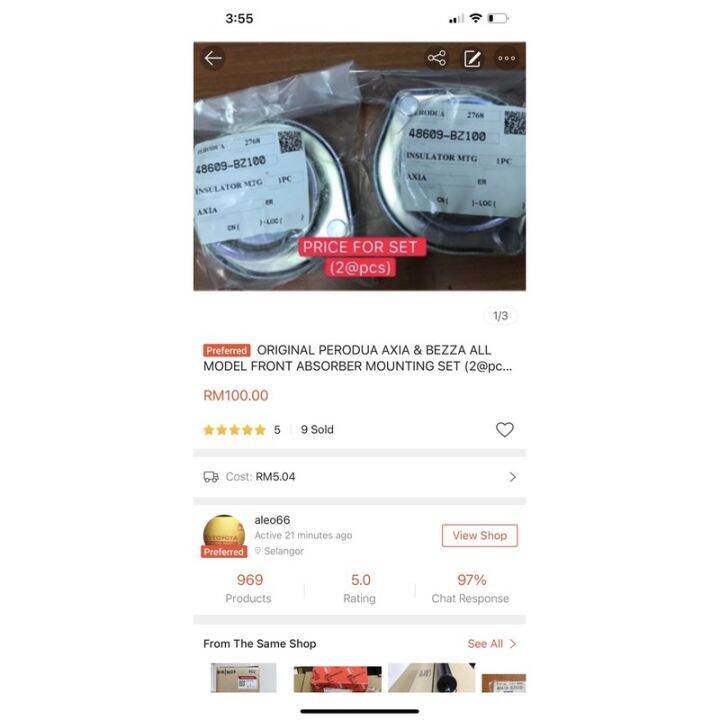This image is a screenshot taken from a cell phone. In the cell phone interface, the upper left corner displays the time as 3:55 against a white background, adorned with black text. The upper right corner shows a signal strength indicator with two out of five bars, a Wi-Fi icon indicating that Wi-Fi is on, and a battery icon. 

Beneath this interface lies a color photograph depicting two metallic components, likely made of stainless steel, encased in a clear plastic bag. These components are positioned side by side on the left side of the image. Each component bears a white label with identical text, which includes a barcode in the upper right corner and reads "Insulator MTG. Axia. One Piece."

Over these labels, the image appears to have been edited to include two red boxes with light red text. The first box contains the text "First price for set," and the box below it reads "Two at PCS."